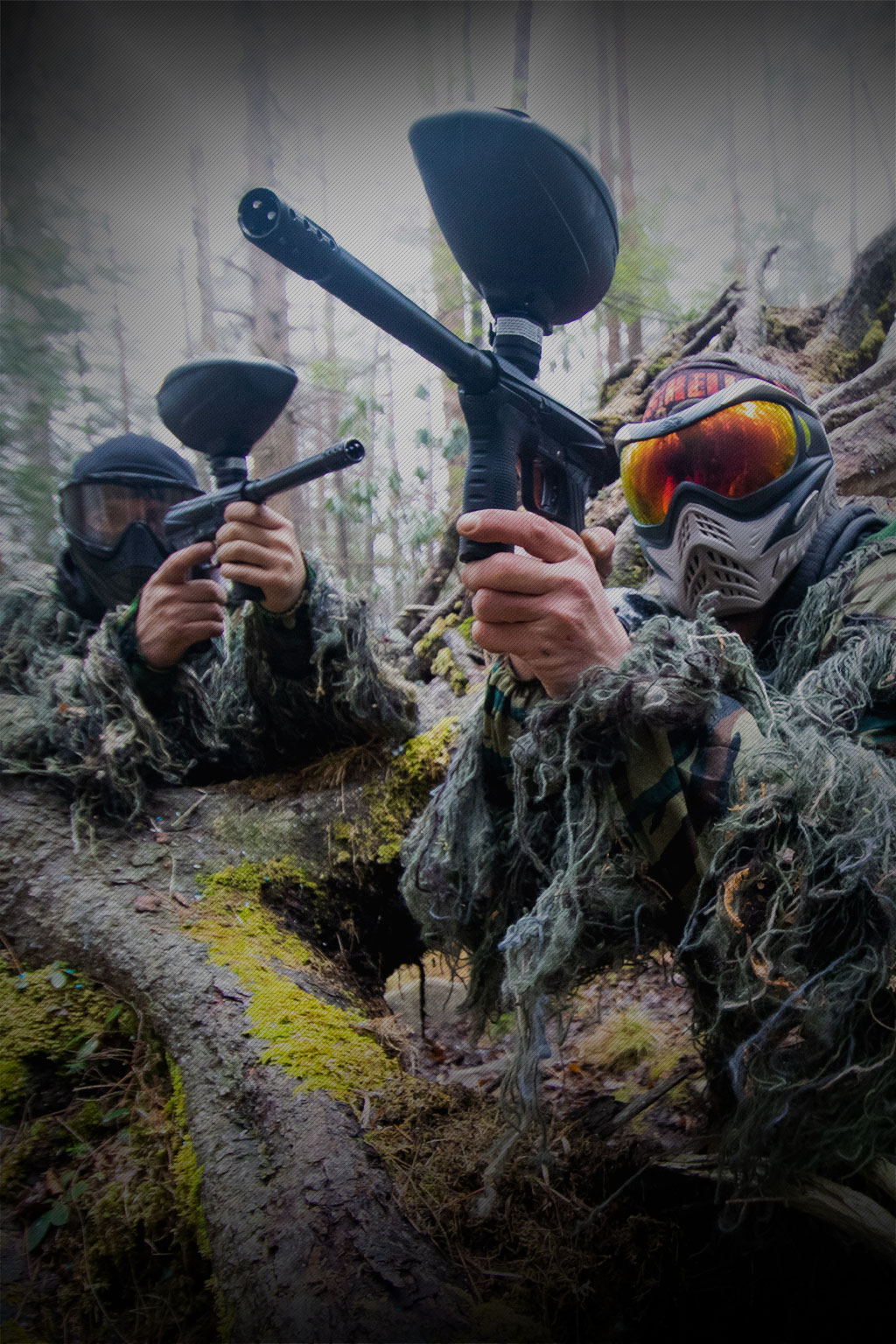In a densely wooded area with tall, thin trees, two men are captured in a color photograph engaging in a paintball game. They are dressed in elaborate camouflage gear, complete with strings of material designed to blend seamlessly with the forest foliage. Both men are lying on a large, moss-covered fallen branch, adding to their concealment. Their faces are fully covered with head cloths, eye goggles, and face masks, leaving only their hands exposed. Each holds a black paintball gun equipped with a top-mounted drum. Positioned side by side, they aim their guns diagonally, the man on the left pointing right and the man on the right pointing left. The barren trees in the background suggest a winter setting, enhancing their camouflaged appearance amidst the stark landscape.